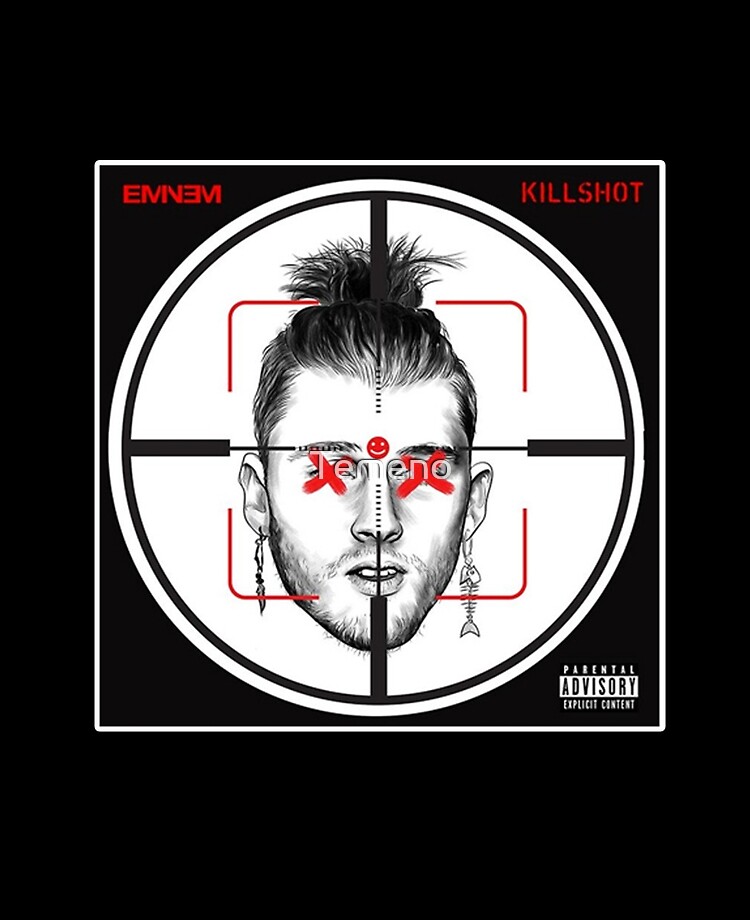The image appears to be an album cover set against a solid black background. The larger frame is a vertical rectangle, with the album cover itself forming a central square. This square album cover also primarily features a black background, with a prominent white circle nearly reaching its edges. The circle contains a black crosshair pattern, creating a narrow white border around it. At the focal point of the crosshairs is a line drawing of a young man with a top knot, five o'clock shadow, and dark hair. The man's eyes are marked by two red X's, and a small red smiley face is placed between his eyes at the center of his forehead. Additionally, he has distinctive earrings; one shaped like a dead fish, and the other resembling bones. In bold red letters, the album title "Eminem Kill Shot" is printed across the top, with a "Parental Advisory Explicit Content" warning located in the lower right-hand corner of the square.